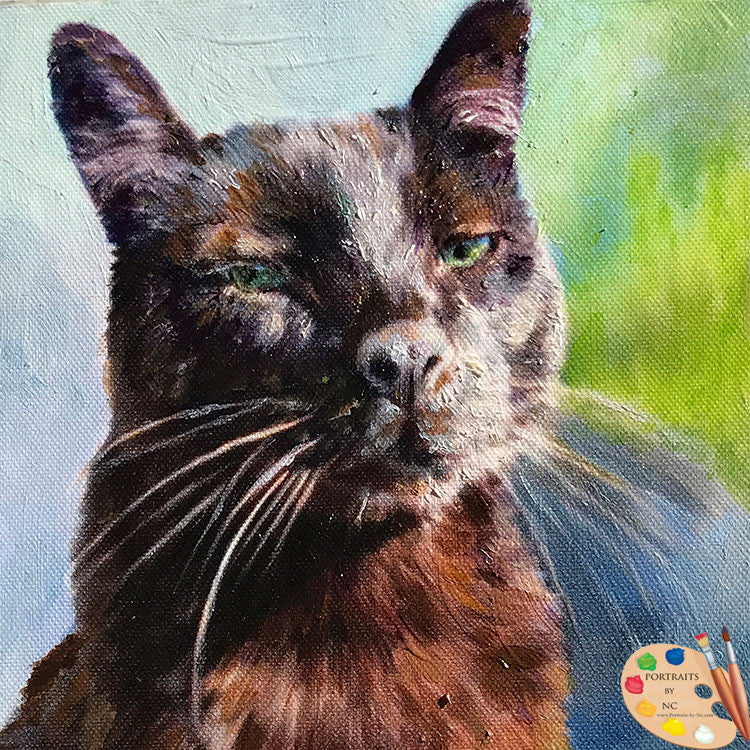This square-shaped painting depicts a front-facing cat from the shoulders up, with its head tilted slightly to the left, occupying a central but slightly left-of-center position in the image. The cat's face and upper body feature a mix of brown, black, and white fur, with its body highlighting some blue hues where the light hits. Its striking eyes, vividly colored in blue and green, are half-closed in a watchful gaze. The cat's fur alternates with brown and orange at the bottom, and it has long, delicate white whiskers. The background of the painting is a blend of light, pale blue on the left, fading into a more vivid green on the right, with an overall abstract and blurry texture that enhances the focus on the cat. In the bottom right corner of the image, there is a palette logo adorned with rainbow-colored paint spots and two brushes, inscribed with the text "Portraits by NC."